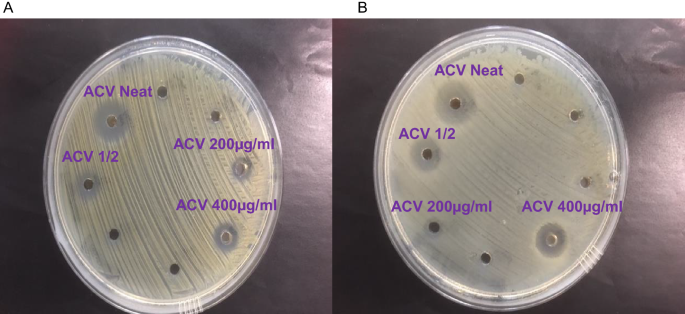This scientific image consists of two labeled sections, A on the left and B on the right, both showcasing growth media plates designed to test fungal growth. Each plate features eight dots, some encircled by clear rings and others appearing as dark black spots. The dots are consistently labeled with "ACV neat," "ACV 1.5," "ACV 200 µg/ml," and "ACV 400 µg/ml." Section A shows some text positioning variations compared to Section B. While Section B's dot labeled "ACV 200 µg/ml" is located on the lower left side of the plate, in Section A, it is positioned on the upper right side. The plates themselves are clear, and the labeling text is predominantly purple. The background is a black laboratory surface, enhancing the distinct visibility of each test spot.